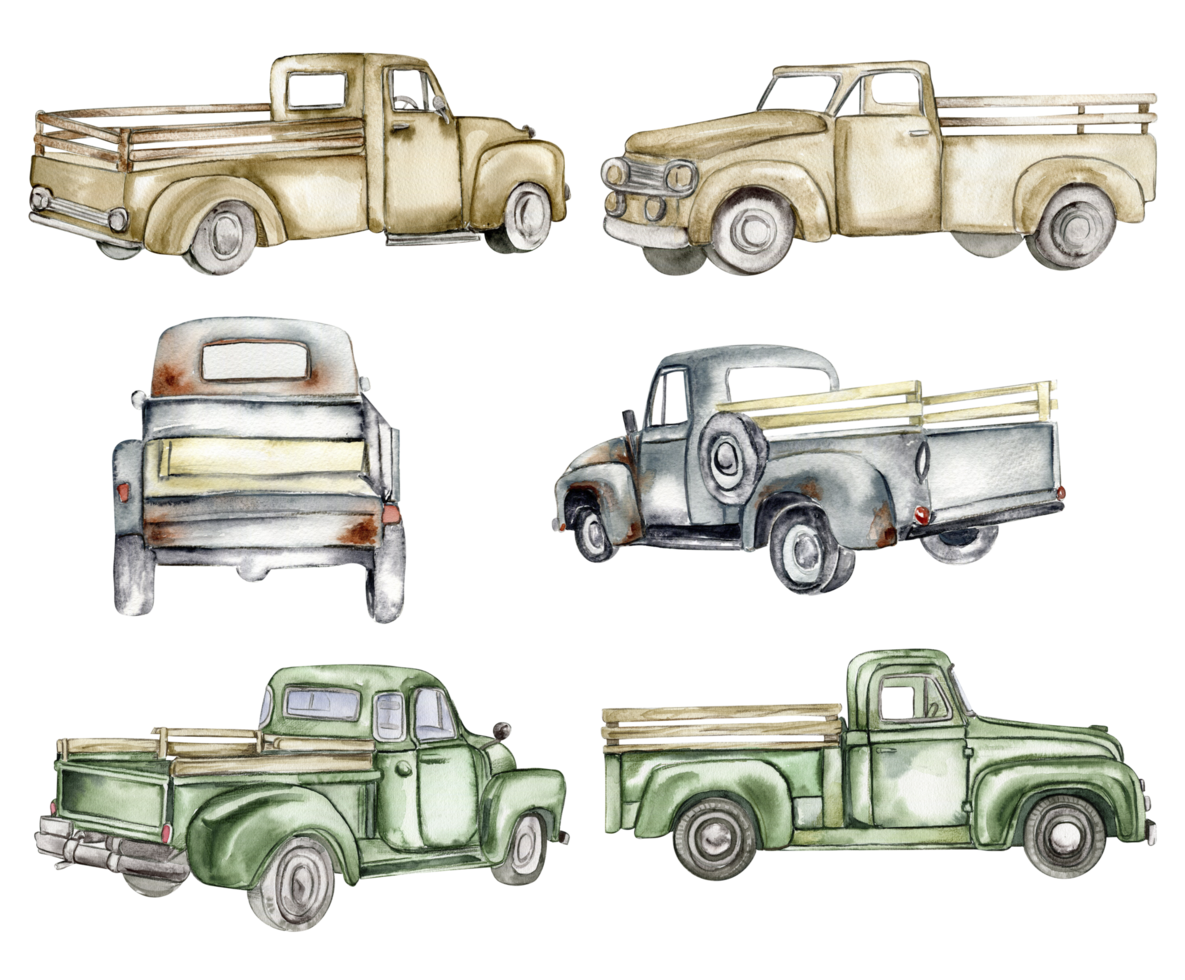The image features six detailed watercolour paintings of vintage 1940s pickup trucks, arranged symmetrically in two columns and three rows. Each truck is depicted from different angles, showcasing the right side, left side, and backside views for a comprehensive visual understanding. 

In the top row, there are two light brown trucks. The one on the left displays the right side and rear of the truck, while the one on the right shows the front and left side. Moving to the middle row, the trucks are a bluish-grey hue, each adorned with red markings. The left painting reveals the rear side, complemented by a wooden section behind the truck, whereas the right displays the left side, featuring a spare tire positioned just behind the driver's door. Finally, the bottom row presents green trucks with a minimalist design, showing primarily boards on the left and right sides. The left painting in this row provides a view of the back and left side, while the right one offers a perspective of the truck's right side. 

Subtle differences in rear windows, side view mirrors, and cab designs highlight variations across these otherwise similar-looking vehicles, adding dimension and detail to the artwork.